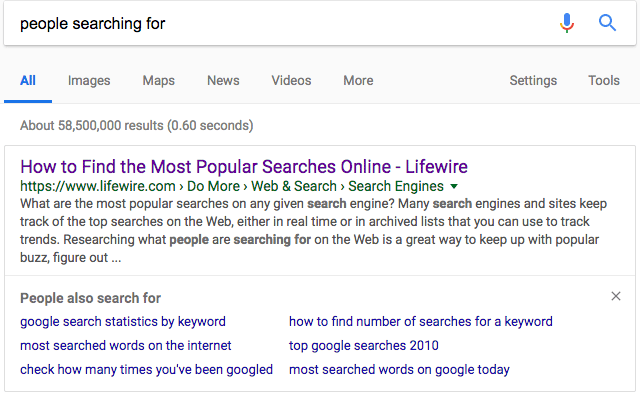An image showing a screenshot of a Google search results page. At the top, there is a search bar with the text, "people searching for our microphone magnifying glass blue," indicating the search query used. The page displays several tabs below the search bar, including Images, Maps, News, Videos, More, Settings, and Tools. 

Just below these tabs, text indicates there are approximately 58 million results for this query, retrieved in 0.60 seconds. The first search result is highlighted in purple and reads, "How to Find the Most Popular Searches Online - Lifewire," with a URL starting with "https://..." 

The result snippet elaborates on the topic, explaining how various search engines track the most popular searches, either in real-time or through archived lists, and how this data can be used to track trends and understand what people are searching for online. Additional related searches and suggestions are listed, including phrases like "Google search keyword," "most searched words on the internet," "check how many times you've been Googled," "how to find the number of searches for a keyword," "top Google searches 2010," and "most searched on Google today."

The dense and detailed content reflects the practice of tracking and analyzing popular search queries to stay informed about current online trends.